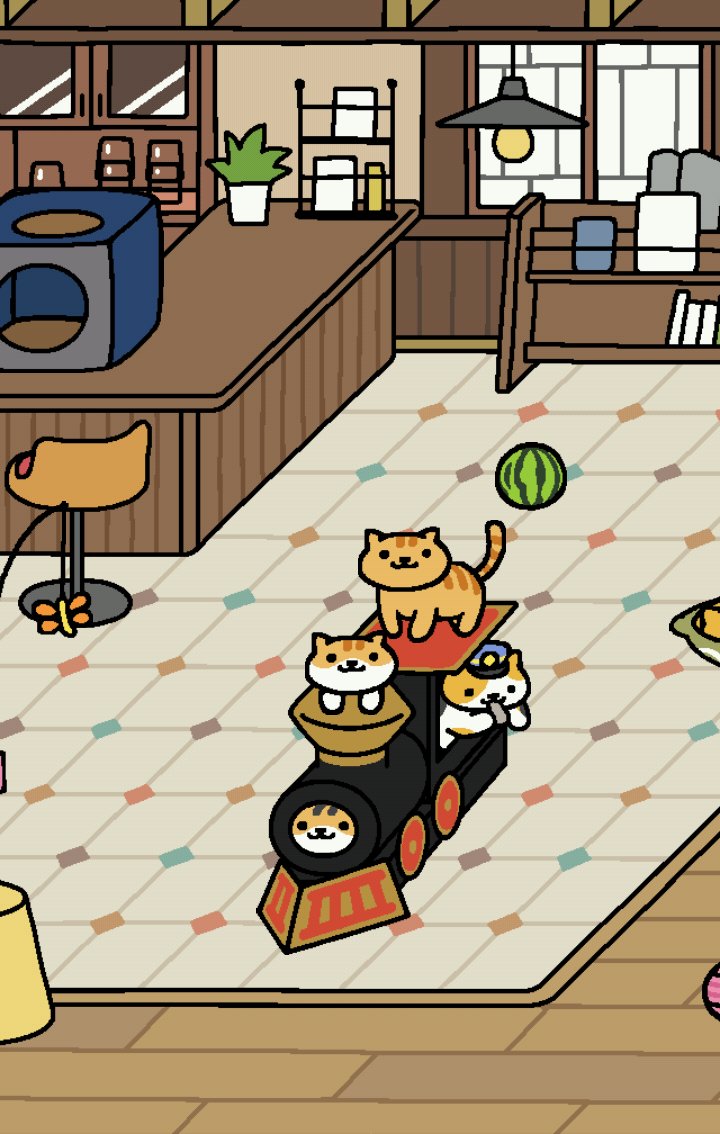In this detailed, digital art screenshot from the mobile game Neko Atsume, a charmingly illustrated indoor bar area is depicted. The environment features a wooden counter with an orange stool in the top left corner, next to a magazine rack. Both are set against a backdrop of Japanese-style walls and windows. Below, a tan tile floor, divided into squares by multicolored diamonds in teal, orange, pink, and brown, adds a playful element to the scene. On the counter, there's a white plant vase with green foliage and a blue cube with circles. Adjacent to these items, wooden shelves hold various books and items, adding to the cozy interior.

In the foreground, a whimsical, cartoon-style black model train with red and gold accents forms the centerpiece. This toy train hosts four adorable cats: one cat dressed as a conductor peeks out from the side window, blowing a whistle; an orange tabby stands on the train’s red roof, looking directly at the viewer; another cat, with an orange tuxedo-like pattern, sticks its head and paws out of the chimney pipe; and the fourth cat, with an orange and white face, occupies the front of the train. The cats are drawn with simple but charming details: thick black lines, dot eyes, tiny noses, and small mouth lines, perfectly capturing the playful and endearing essence of Neko Atsume.